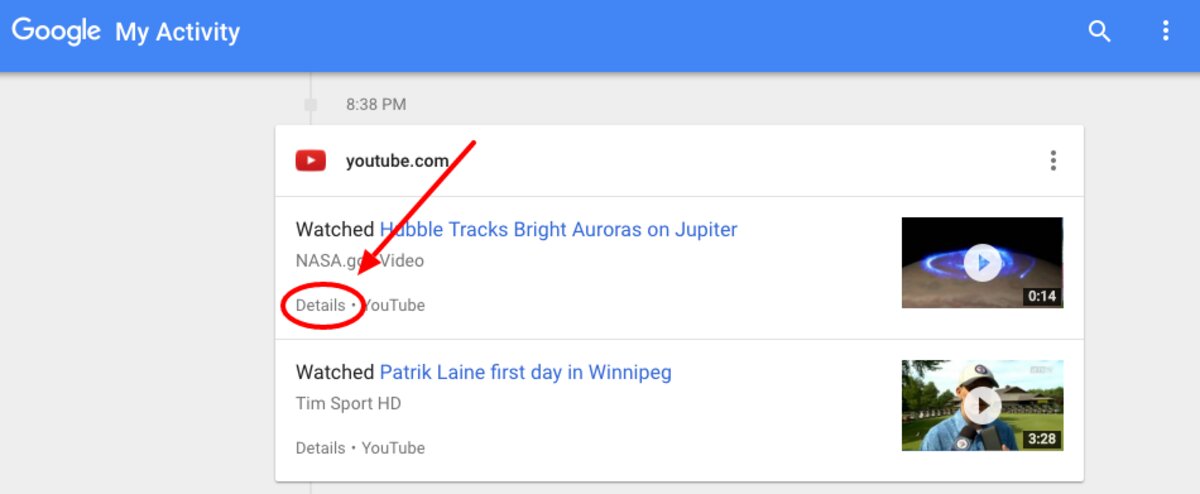This image is a screenshot of a Google My Activity page, prominently featuring a large horizontal blue bar at the top. In the upper left corner of this bar, the white Google logo is displayed alongside the title "My Activity." On the top right, there is a white magnifying glass icon, used for searching the activity, and a vertical ellipsis icon, which opens setting options for the page.

Beneath the blue bar, the main section of the page features a light gray background containing a central white box. This white box details the user's recent YouTube activity. At the top of this box, a timestamp reads "8:38 PM." To the left, the red YouTube logo and the text "YouTube.com" signify the source of the activity.

The content of the white box records two YouTube videos that the user has watched: "Hubble Tracks Bright Auroras on Jupiter" and "Patrick Lane First Day in Winnipeg." Each entry includes details such as gray text descriptions and clickable links for directly rewatching the videos. Additionally, the right side of the box showcases the YouTube thumbnails for both videos. The first thumbnail depicts a space scene, while the second features an image of Patrick Lane. Underneath each thumbnail, the video's duration is indicated: the first video lasts 14 seconds, and the second runs for 3 minutes and 28 seconds.